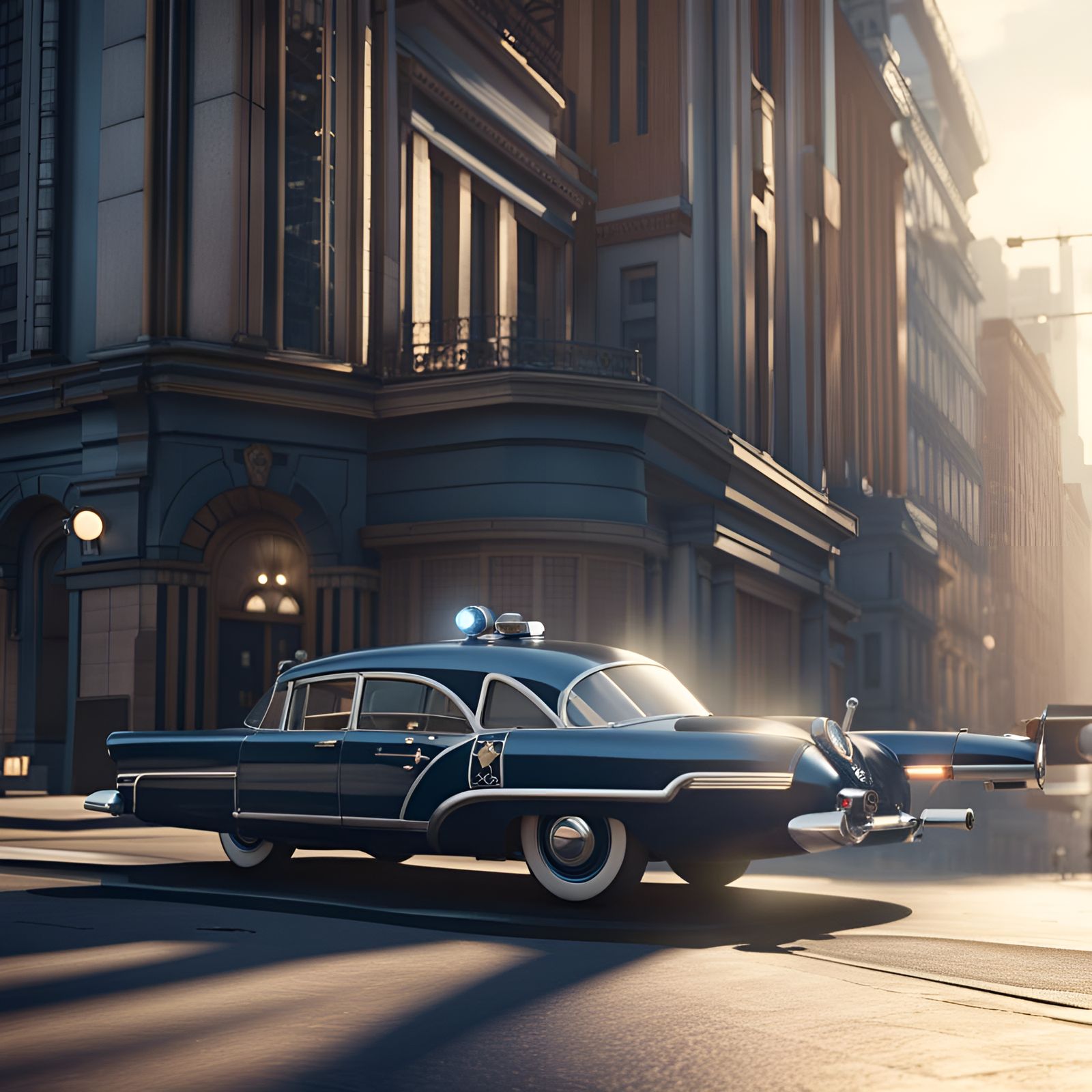The image showcases a 3D generated, shiny, vintage-style police car driving on a concrete road. This dark blue car, reminiscent of designs popular in the 1940s or 1950s, features a small circular light on its roof, likely functioning as a siren. Notable details include silver pipes at the rear and white rims on the wheels, with a clear shadow cast on its left side due to the sun's position. Dominating the background, a large building extends from the street level to the top of the picture, characterized by a grand doorway with lights, a central balcony, and imposing columns that reach the roof. Surrounding this primary structure are other residential and commercial buildings, contributing to a typical cityscape backdrop.